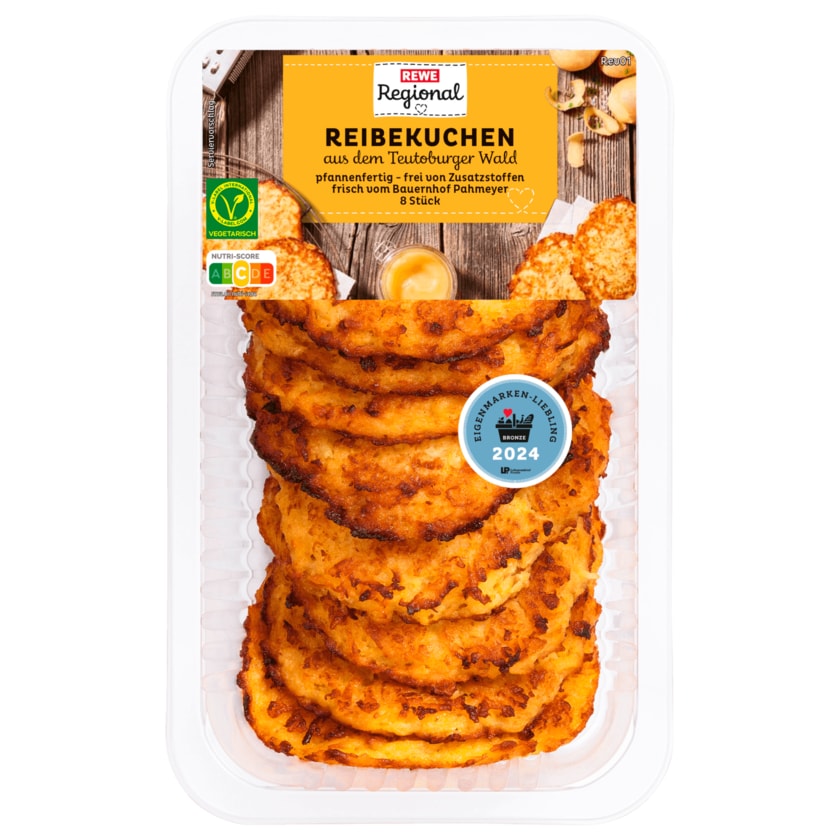This is a detailed photograph of a packaged food product, likely German, by the brand "Rewi Regional." The product, named "Riebeckkuchen," is contained in a clear, translucent plastic deli container with rounded edges, set against a white background. The main label is orange with additional smaller labels in the lower-left corner. The label, mostly in a foreign language, features a green square icon indicating the product is vegetarian. The label image includes a display of the food item, which seems to be meat-like patties or possibly hard-boiled eggs, alongside a metal cheese grater or food grater in the left-hand corner. The packaging rests on a brown wooden surface, adding rustic appeal to the presentation.